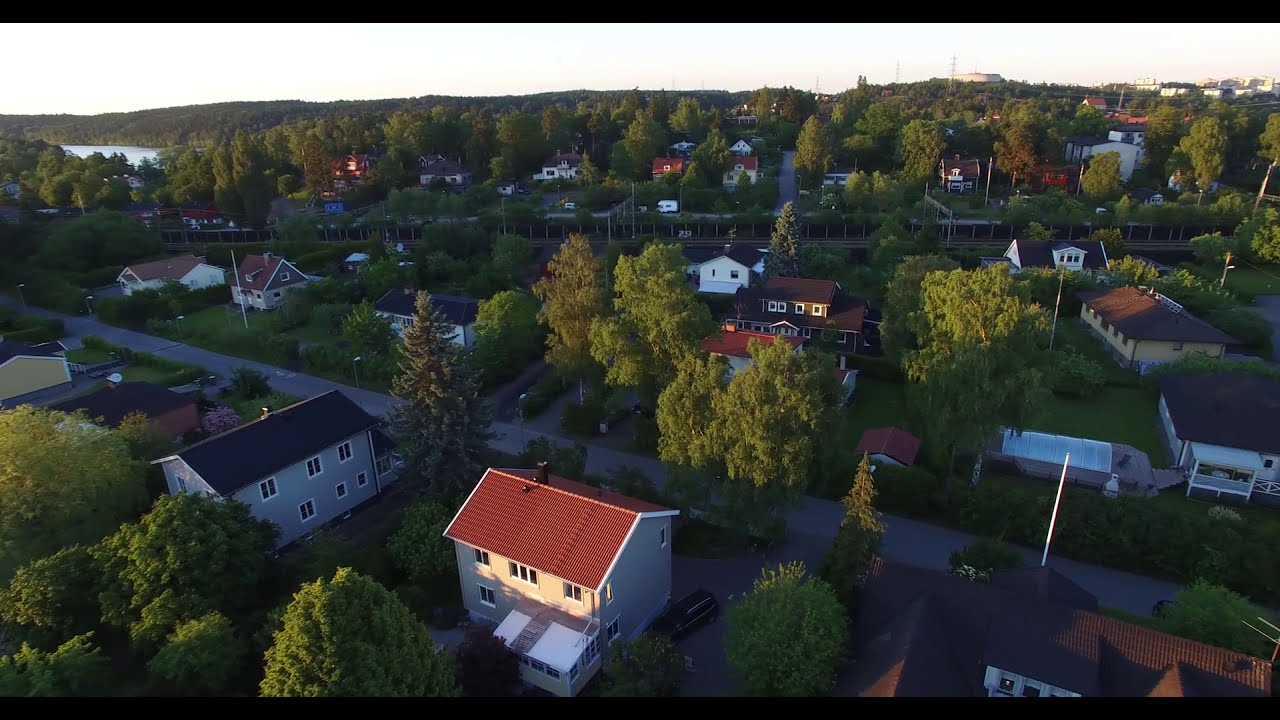The image is an overhead photograph of a sprawling, heavily treed suburban neighborhood, likely established around 50 years ago. The houses come in various sizes, from one to possibly three stories, and are painted in different hues such as gray, tan, white, and beige, with a range of roof colors including red, black, gray, and brown. Among the houses, noticeable ones include a house with a striking red roof and another with blue sides and a black roof. There's also a greenhouse visible in one yard, alongside distinct white and yellow houses.

A road meanders diagonally from the left center to the bottom right of the image, lined with houses and flanked by streetlights. Another roadway or possibly a train track crosses the center of the photograph. In the upper left-hand corner, a large body of water, possibly a lake, suggests this could be a community of lake houses. The abundant tall trees add to the dense, green canopy over the neighborhood. The horizon is visible with a warm, white sky indicating a bright, sunlit or late afternoon setting. A hill in the background hosts what appears to be a plant or factory, adding to the landscape's layered complexity. The photograph is marked by a large black bar at the top, potentially indicating the edge of the frame or an editing artifact.